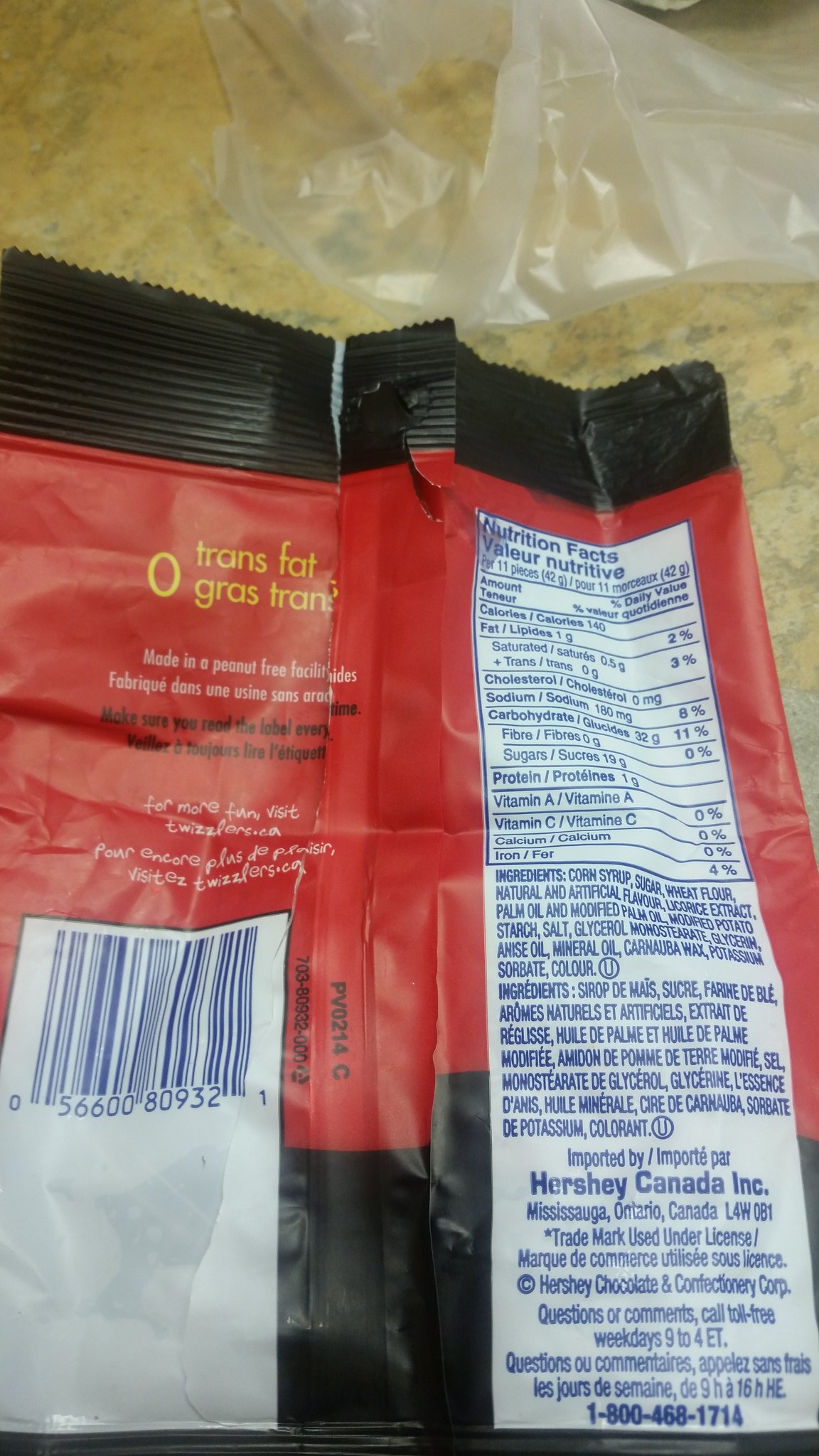The image displays the back of an opened snack bag, prominently featuring a vibrant red body with black horizontal strips at the top and bottom. The red of the bag is contrasted by several white rectangles: one on the left with a navy barcode and numbers, and another on the right displaying the nutritional facts in dark blue print. Notably, the package boasts "Zero Trans Fat" in yellow lettering against the red background, alongside various details about the snack, such as ingredients like corn syrup, sugar, and wheat flour. The crumpled bag, indicative of a corn snack, rests on a yellowish granite counter. Above the crumpled snack bag, an open clear plastic bag is also visible. At the very bottom of the package, a navy-blue phone number, 1-800-468-1714, can be seen, along with trademarks and information indicating it is imported by Hershey Canada.